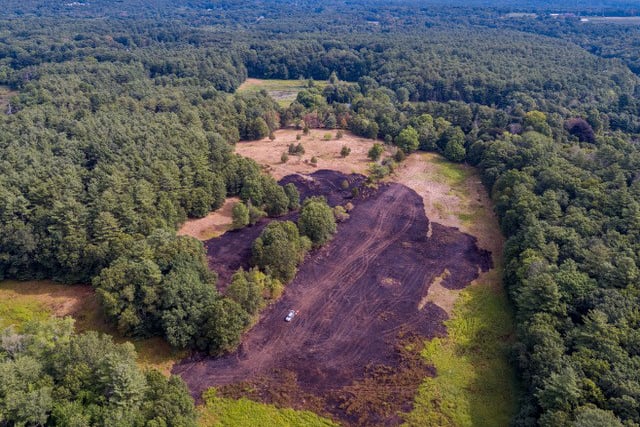This aerial photograph captures a vast, dense forest, with hundreds upon hundreds of dark, towering trees stretching as far as the eye can see. In the midst of this sea of green foliage is a prominent clearing, its ground appearing worn and scattered with tire tracks. This open area features patches of brown dirt and a darker section that resembles an oil spill or possibly a marked zone, giving the impression of an unusual coloration. At the bottom center of the clearing sits a solitary white vehicle, possibly an SUV, oriented towards the bottom left of the image. The vehicle is set against a contrasting backdrop of light and dark greens, with hints of both white road tracks and peculiar purple hues that obscure part of the land and some trees. In the far distance to the right, near the top edge, a structure resembling a house can be vaguely seen, faintly blending into the forested landscape.